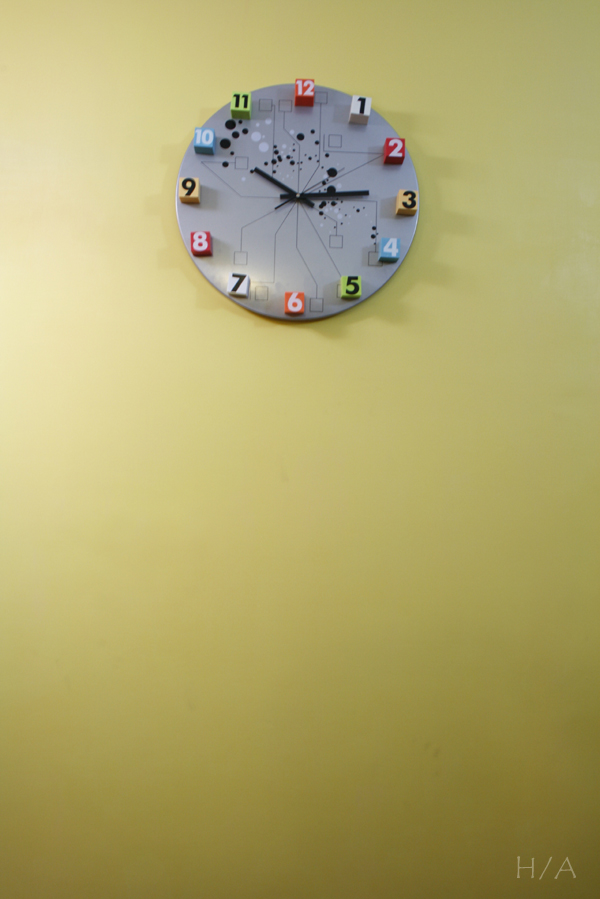This vertical image features an unusual, wall-mounted clock prominently displayed on a greenish-yellow wall. In the lower right corner of the image, the initials "H/A" are inscribed in light green. 

The clock is gray, seemingly made of plastic, and has a distinctive dome shape. The clock face is adorned with three-dimensional numbers, varying in color between black and white in an alternating pattern. Starting from the white "12" at the top, the sequence continues around the clock face until reaching the black "11." The hour and minute hands are both black, as is the second hand.

Adding to the clock's unique design, black lines emanate from the center of the clock, extending outward toward each hour. These lines feature various intricate symbols, including squares and stars. Additionally, the upper left section near the center of the clock is sprinkled with small black and gray circles, enhancing its quirky visual appeal.